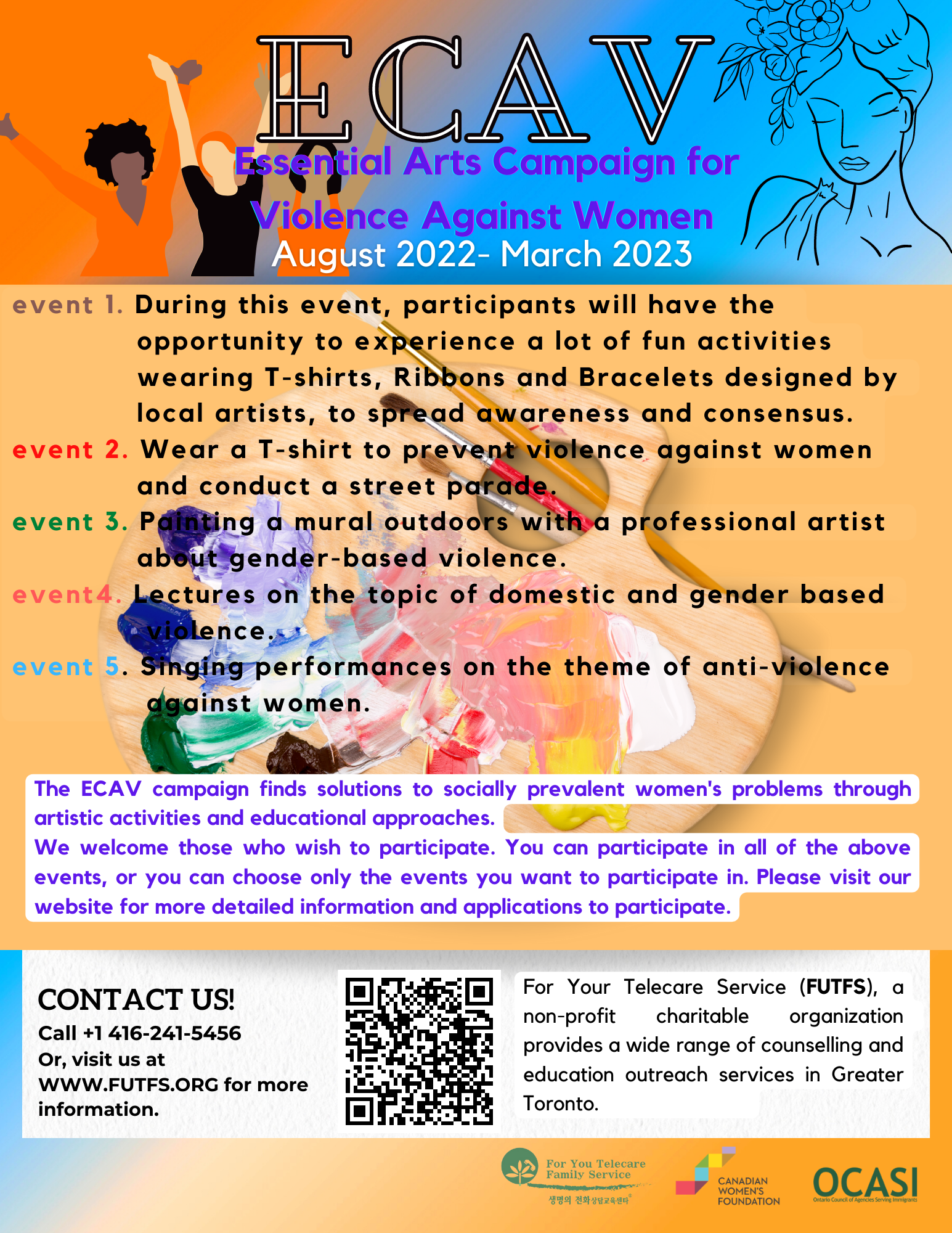This image is an event poster for the ECAV (Essential Arts Campaign for Violence Against Women) running from August 2022 to March 2023. The header at the top showcases the ECAV title in a fancy white font with a black outline against a gradient background transitioning from orange to blue. 

On the left side of the header, there are three non-descript cartoon women with their arms raised in celebratory poses, while the right side features a detailed black outline illustration of a woman wearing a headdress made of flowers and dressed in a toga, visible up to her chest.

The middle section of the poster includes a list of five events, each detailed with colorful text. Event One highlights fun activities where participants can wear T-shirts, ribbons, and bracelets designed by local artists to spread awareness. Event Two involves wearing a T-shirt to prevent violence against women and conducting a street parade. Event Three focuses on painting a mural, Event Four offers lectures on the topic, and Event Five features singing performances on the theme.

Beneath the list of events, there's an informative blurb in purple text over a white background that states, "ECAV Campaign to Find Solutions to Socially Prevalent Women's Problems Through Artistic Activities and Educational Approaches. We welcome those who wish to participate."

At the bottom of the poster, the center features a QR code. The lower left contains contact information, and the lower right includes logos of various sponsors. The design is aimed to be visually appealing for social media and print distribution.